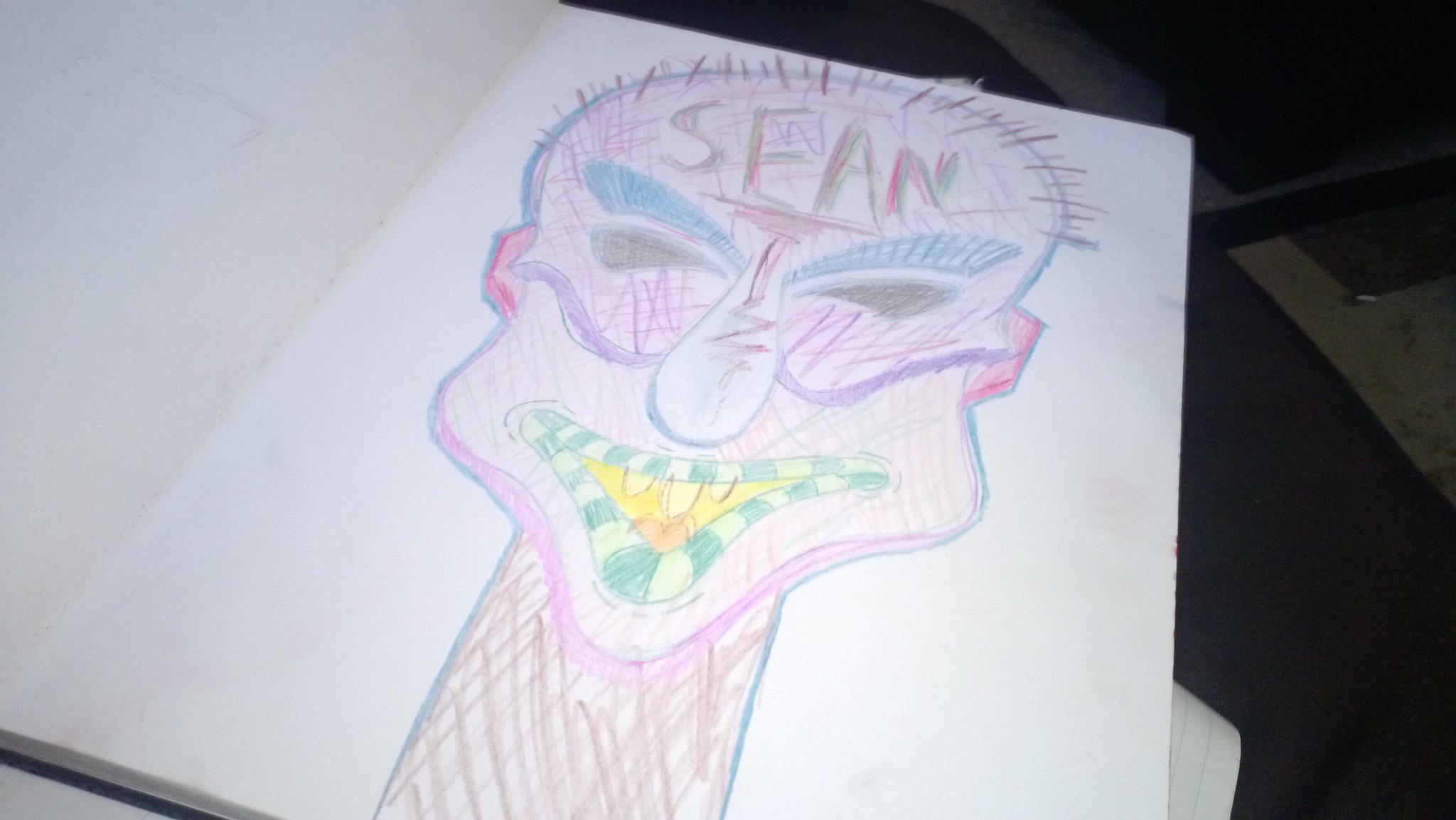This image is a vibrant and exaggerated colored pencil drawing on a large page of what appears to be an art book. The subject is a surreal and cartoonish face with the name "Sean" inscribed in red and brown on the forehead. 

The character has distinct blue eyebrows with smaller black eyes positioned below them, giving a quirky expression. The nose is teardrop-shaped and white, contrasting sharply with the surrounding colors. The mouth features striking green and yellow striped lips, containing a yellow interior and a visible tongue at the bottom, along with three protruding teeth.

The head has a rounded shape with disheveled brown hair sticking out. Its ears are vibrant red, adding to the whimsical feel. The chin has an unconventional, exaggerated shape, leading the sides of the face to flare out at the cheekbones before tapering to a point at the lips, which mirror the same pointed structure.

The neck is elongated and outlined in blue, filled with brown cross-hatchings that add texture. The skin of the face is primarily pink with blue lines running under the eyes, almost resembling the bottom edge of a mask. There are also light purple scratchy markings scattered across the face, adding to the abstract and unfinished aesthetic. The head itself is a mix of purple and brown hues, creating a sense of depth and complexity.